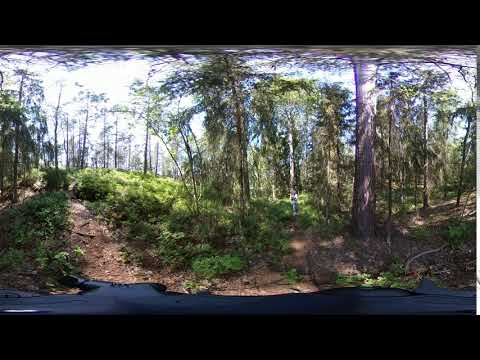The image is set in a lush forest, characterized by its verdant green undergrowth and tall, imposing trees. There's a particularly massive tree positioned to the right side of the scene, creating a focal point among the smaller trees and green shrubbery surrounding it. Multiple dirt paths meander through the woods, offering a sense of exploration and tranquility. The paths are lined with green and brown hues, while shadows and light interplay to create a serene atmosphere. In the middle distance, a person can be seen walking along the path, dressed in a white shirt and jeans, emphasizing the human connection with nature. The image appears slightly distorted, likely due to being taken with a wide-angle or 360-degree panoramic camera, which causes the straight lines to curve and enhances the expansive feel of the scene. The photograph captures a moment of simple, serene beauty in the woods, potentially inviting a hiker or mountain biker to lose themselves in its tranquility. The scene is sunlit, indicating it has been taken during the daytime, with light filtering through the trees, highlighting the natural beauty of the forest setting.